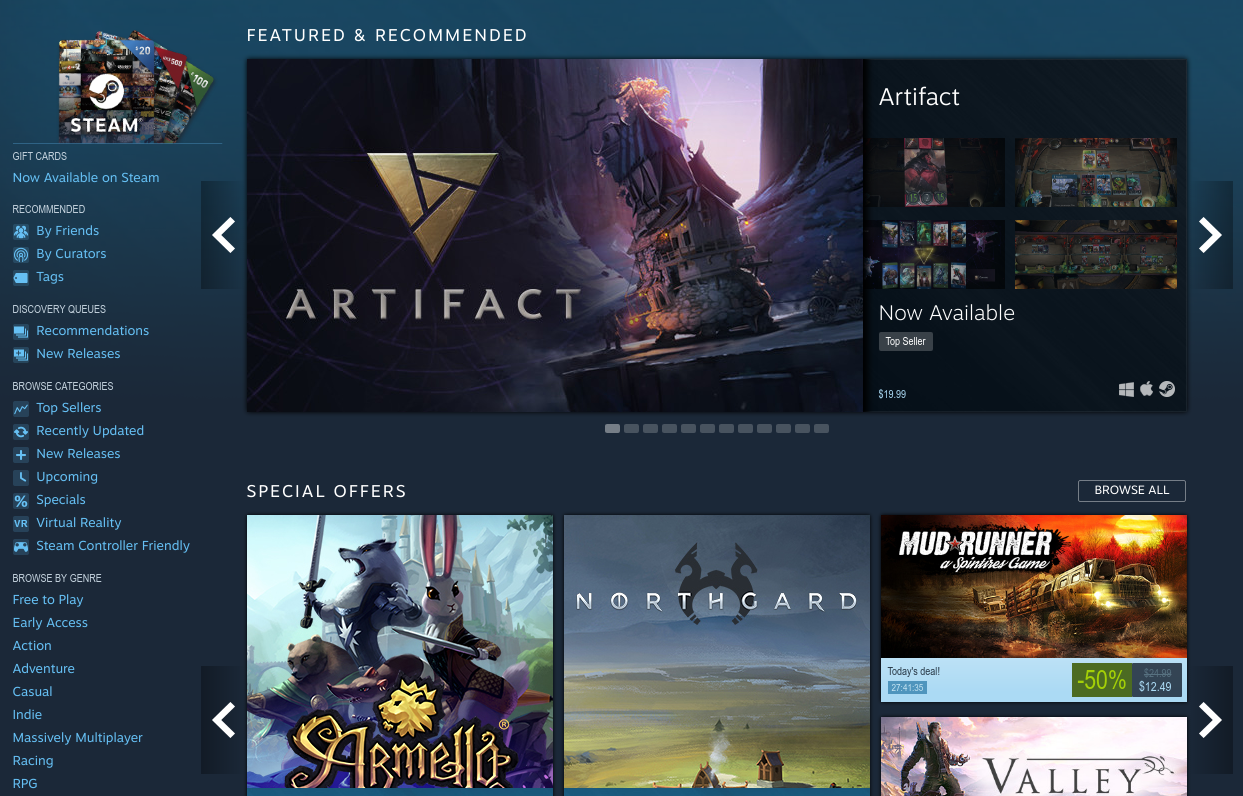**Detailed Caption:**

This image depicts the Steam interface featuring a variety of sections highlighting games and special offers. In the top left corner, the Steam logo is prominently displayed, with accompanying Steam cards and prices below it. To the right, the section titled "Featured and Recommended" in white lettering introduces a spotlighted game. The featured game here is "Artifact," showcased with its distinctive golden triangle logo. The game's artwork depicts a dilapidated house nestled within a snowy valley, suggesting an intriguing setting. 

On the right side of the featured game, additional images and graphics indicate that "Artifact" is a card-based game. The labels "Now Available" and "Top Seller" alongside a price of $19.99 emphasize its market status. 

Below the featured section, the "Special Offers" area displays several highlighted games. On the left, "Armello" is shown with its vibrant cover art featuring various anthropomorphic animal characters wielding swords against a castle backdrop. Next to it is "Northgard," illustrated with a serene field and quaint houses. To the right of "Northgard" are the titles "MudRunner" and "Valley," each represented with their respective visual covers.

On the left-hand side of the interface, the navigation panel lists various interactive links including categories like "Recommended," "By Friends," "By Curators," and "Tags." Additional sections such as "Discovery Cues," "Browse Categories," and "Browse by Genre" provide further exploration avenues within the Steam application.